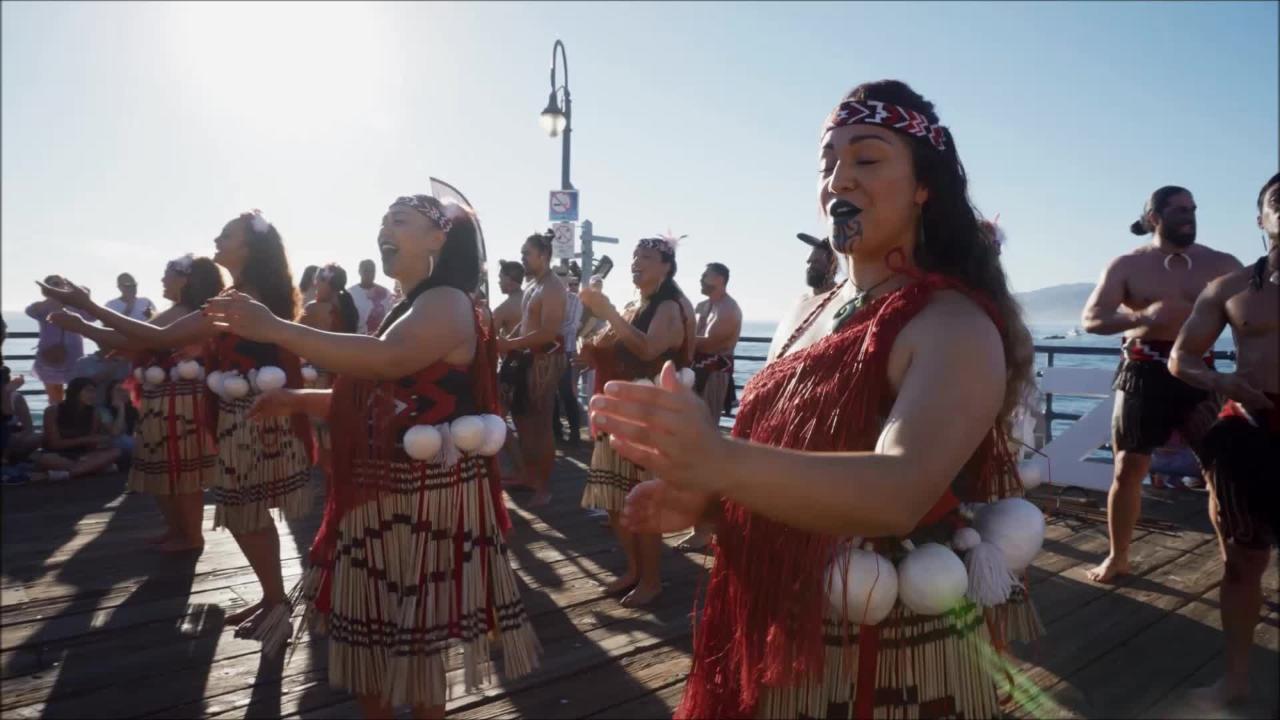The image captures a group of Pacific Islander performers, likely of Samoan or Maori descent, engaged in a traditional dance or haka. In the foreground, four women are visibly dressed in elaborate tribal attire. They wear red, one-shouldered tops adorned with fringe, and intricate jewelry. Their waist belts are decorated with large white balls resembling those made of cloth or string. Below these belts, the women sport grass skirts in tan hues with black geometric accents in the shape of triangles and lines. Notably, the woman leading the group has distinctive tribal tattoos extending from her bottom lip down to her jawline. All the women are barefoot, adding to the authenticity of their traditional ensemble. Behind them, more dancers, both male and female, are dressed in similar tribal outfits, with the men wearing black shorts and shark tooth necklaces. Their hair is pulled back into ponytails, and they are also barefoot. In the distant background, several onlookers, possibly tourists, capture the moment on their cameras, suggesting that the performers are entertaining a crowd. The scene is set on a wooden surface, like a bench or a porch, enhancing the communal and cultural atmosphere.